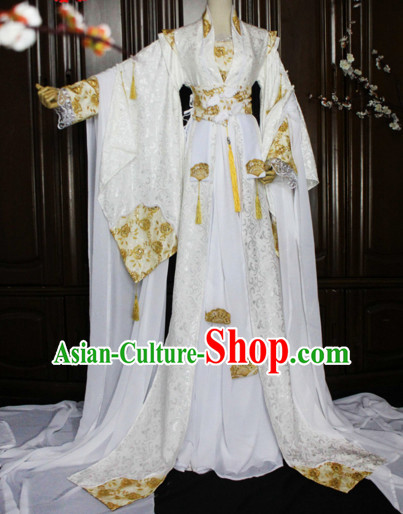In this image, a model or mannequin is adorned in a traditional yet modernized long, white dress with intricate lace and flowing silk fabric. The dress, which extends well past the floor, features metallic gold accents along the edges of the sleeves, hem, and accompanying scarf. The sleeves are notably long and droop elegantly, almost forming a train. The mannequin itself has a white body with gold-painted hands extending to one side. The dress's layered structure presents a mix of white tones, including deeper, darker shades and silvery-whites, with hints of yellow fabric sewn into the hip area. The dress has a v-neckline and is partly overlaid by a mostly gold leather shirt. 

In the foreground, out of focus, are flowers resembling Japanese cherry blossoms, while additional branches are visible in the top left and right corners. The background reveals large, shiny wooden panels, reflecting the flash of the camera. Overlaying the image is text that reads "asian-culture-shop.com," where "asian-culture" and ".com" are in green with a white border, and "shop" is prominently larger and in red.